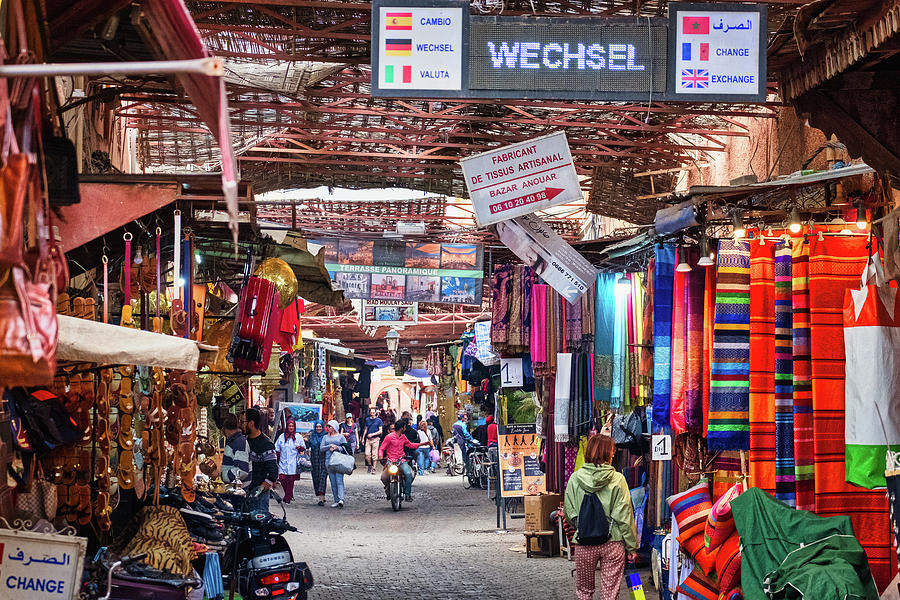The photograph captures a vibrant and bustling open-air bazaar, likely set in an Arab or Middle Eastern country, given the Arabic writing on signs and the diversity of head coverings among shoppers. The market is teeming with activity; people walk through the narrow street, which is also navigated by individuals on mopeds. The scene is richly colorful and detailed. On the right side of the image, there are beautifully dyed fabrics and tapestries hanging, illuminated by overhead lighting, inviting closer inspection from a woman nearby. Across the walkway, a vendor displays a variety of leather sandals. Overhead, a sign for currency exchange services features flags from various countries, indicating a tourist-friendly locale. The bazaar stretches on as far as the eye can see, with a thatched roof providing shelter. Further in the background, an array of different wares and vibrant posters capture the eye, contributing to the overall lively and crowded atmosphere of this foreign market.